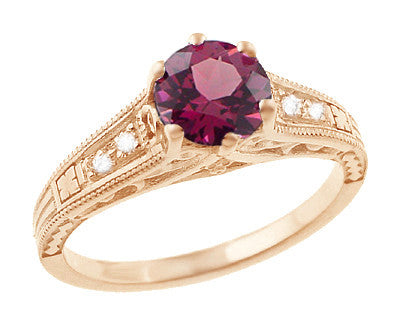This image showcases an intricately designed gold ring set against a plain white background. The ring features a wide, plain gold band that transitions into an ornate, heavily textured front end. The sides of the ring are adorned with four small white gemstones, two on each side, intricately inlaid within the pattern. The main highlight of the ring is a large, well-cut, and sparkling purple gemstone—possibly an amethyst or a purple diamond—situated prominently at the top. The photograph is taken from a slight downward angle, emphasizing the elegant design and luxurious details of the ring.